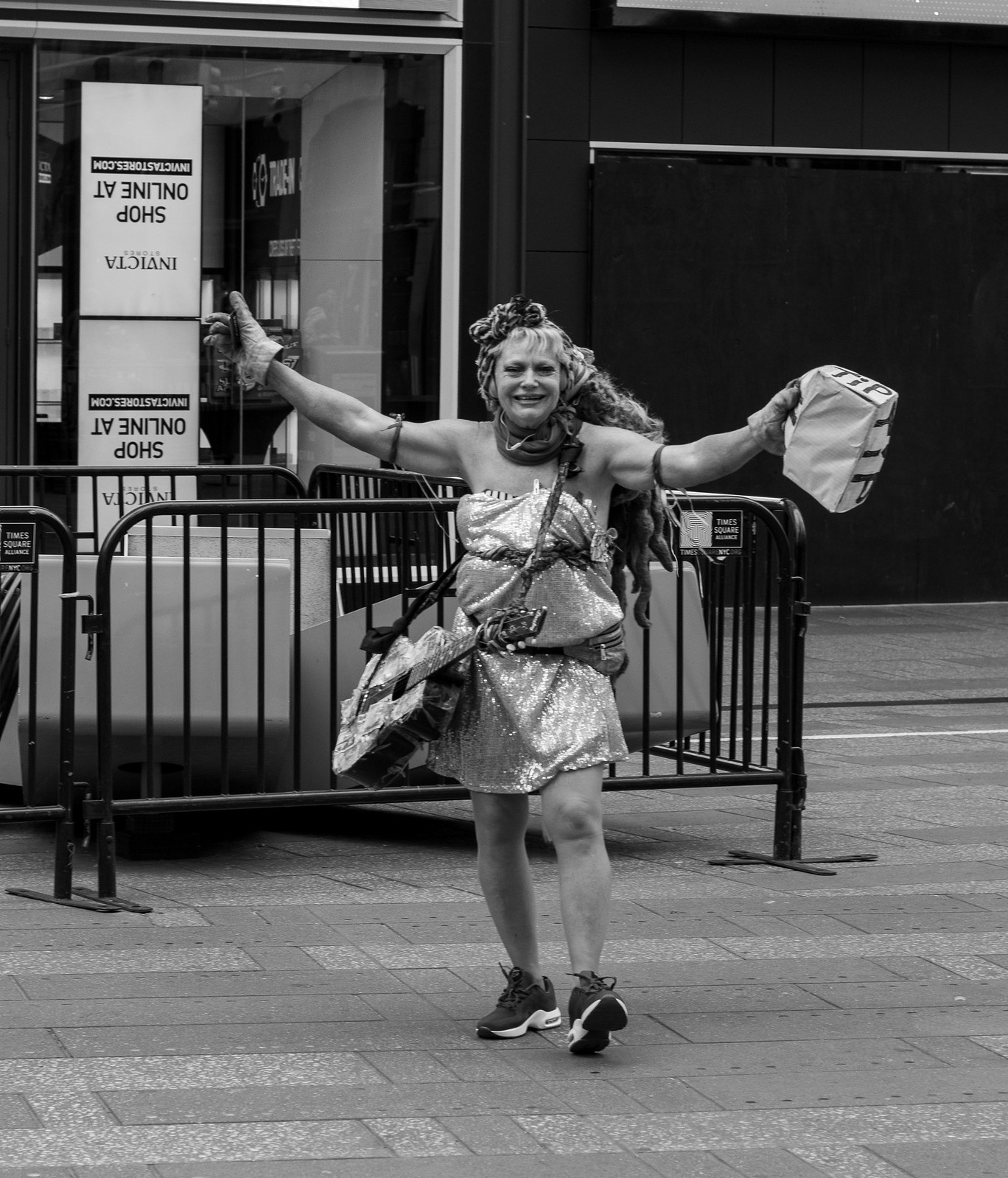In this black and white photograph, a woman stands prominently at the center, framed by an array of details that tell a captivating story. She wears a shiny, sleeveless silver dress with possible clothes pins holding it up, and her long hair, either dreadlocked or simply flowing down her back with bangs, might have a barrette or flowers in it. Around her neck is a scarf, and slung over her shoulder is an acoustic guitar. Her arms are outstretched, each hand clad in heavy leather gloves, and she holds a basket marked with "tip" in one hand. Complementing her outfit, she sports sneakers on her feet.

The background provides context for this outdoor scene. She stands on a sidewalk, flanked by a metal fence and a black barricade, behind which looms a large glass window of a storefront. The window bears signs with upside-down writing, promoting "Invicta shop online at invictastores.com." To the right of the window, a solid black wall contrasts with the reflective surface of the glass, completing the vivid urban backdrop.